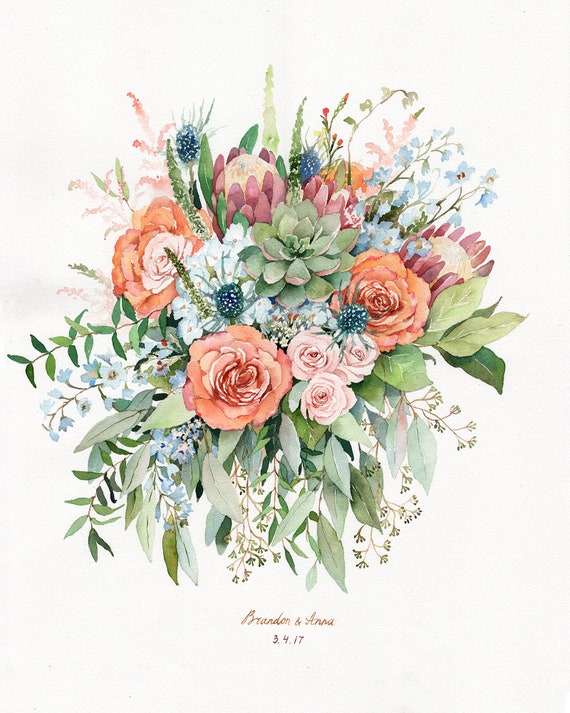This image features a vertically aligned rectangular watercolor painting or drawing with a soft beige or white background. Central to the artwork is a bouquet of diverse flowers and leaves, predominantly showcasing red, coral, and lighter pink roses. The most prominent elements are three large coral-colored flowers and various smaller pink roses scattered throughout. The bouquet is complemented by intricate greenery with leaves of various shapes and shades of green and gray. Blue flowers with small petals and feathery-tipped, narrow, and tall blossoms are delicately interspersed, adding a touch of elegance and variety in color. At the bottom center of the artwork, "Brandon & Anna" is elegantly written in cursive, with the date "3.4.17" below, signifying a significant date, likely their wedding date.